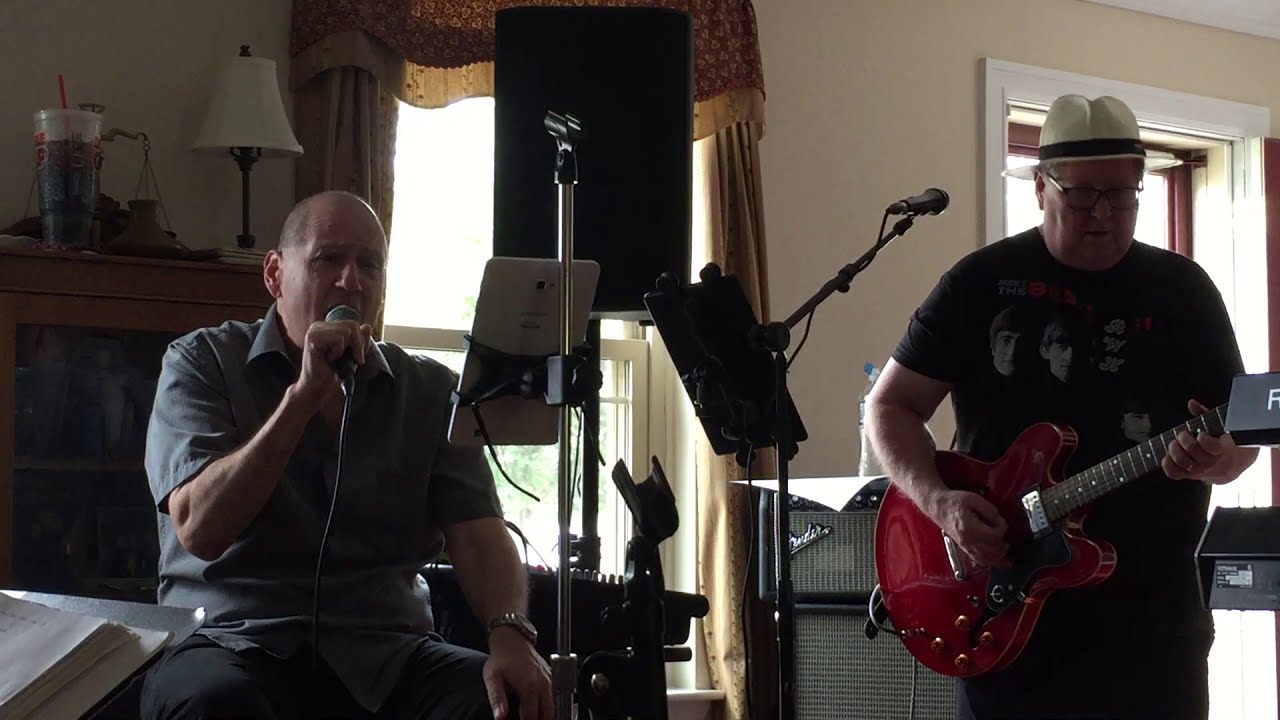The image captures a lively indoor scene where two older men, likely in their late 50s or early 60s, are passionately making music in a cozy room, perhaps a living room. The man on the left, who is bald and dressed in a standard gray zip-up shirt, is seated and holding a microphone to his mouth, possibly singing. In front of him, a mic stand supports a tablet that he uses to read lyrics or music. To his left, just above shoulder height, a Big Gulp soda and a lamp with a white lampshade rest on a surface.

The man on the right is deeply focused, wearing a white fedora with black detailing and a black Beatles t-shirt. He strums a shiny red electric guitar, which resembles a Gibson model. A speaker is positioned behind him, indicating the equipment setup for their practice or performance. The background reveals a window beside a door that has an inset window, allowing daylight to illuminate the scene. Additionally, a fireplace adorned with a drink featuring a red straw further adds to the room's homely atmosphere. The overall setting suggests that the duo might be rehearsing for a future gig or simply enjoying a musical session together.